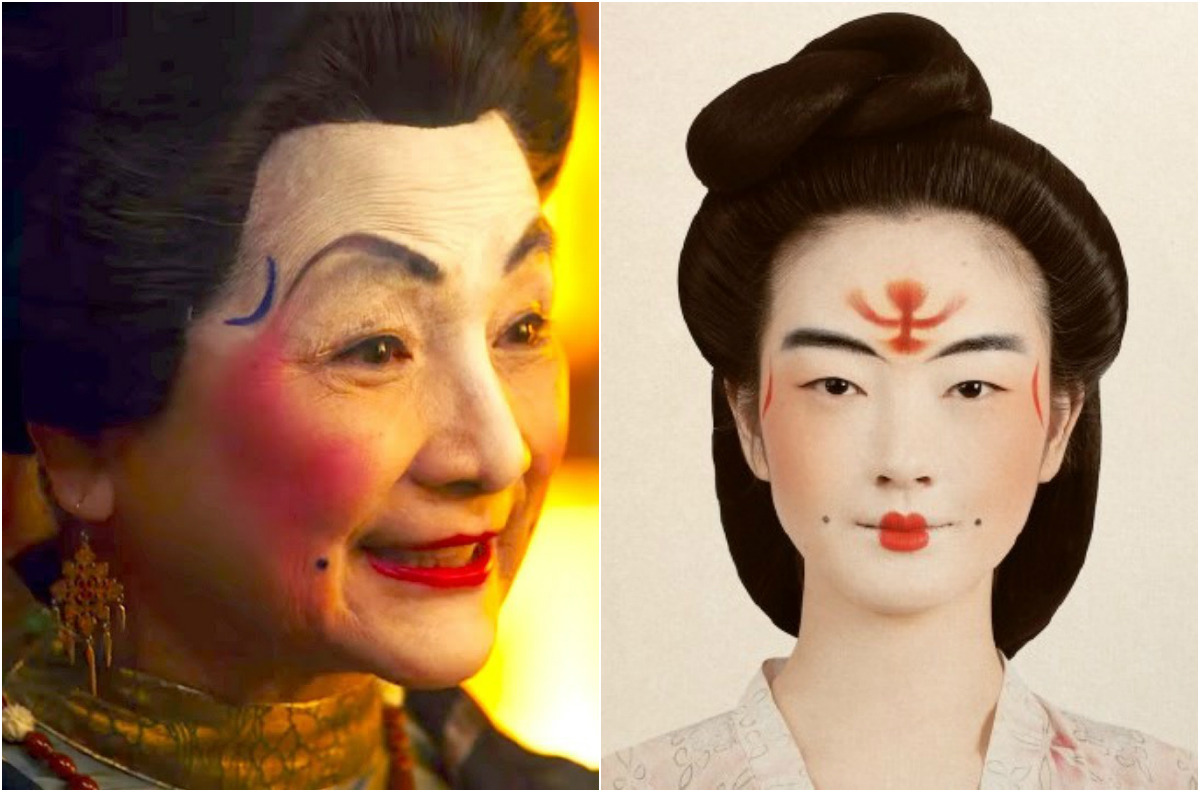Side by side, two women dressed in traditional Japanese costumes grace the screen. The woman on the left, appearing older, sports a distinctive white-painted face adorned with dramatic red lipstick covering her entire lips. A small black mole marks her right cheek, which is heavily blushed in red. She wears a gold earring and a red necklace, complemented by a gold collar on her shirt. Her hair, seemingly a wig, is combed back neatly, with a striking blue slant marking above her right eyebrow.

To the right, a younger woman stares directly into the camera. Her face is also painted white, accentuated with bright red lipstick. A prominent red emblem or logo decorates her forehead, contrasting with her dark, sleek hair pulled back into a bun. She is dressed in a white V-neck robe adorned with a subtle flower pattern. The backdrop behind her is a soft cream color, which enhances the vividness of her makeup and attire. Together, these images capture the essence of traditional Japanese style and elegance.